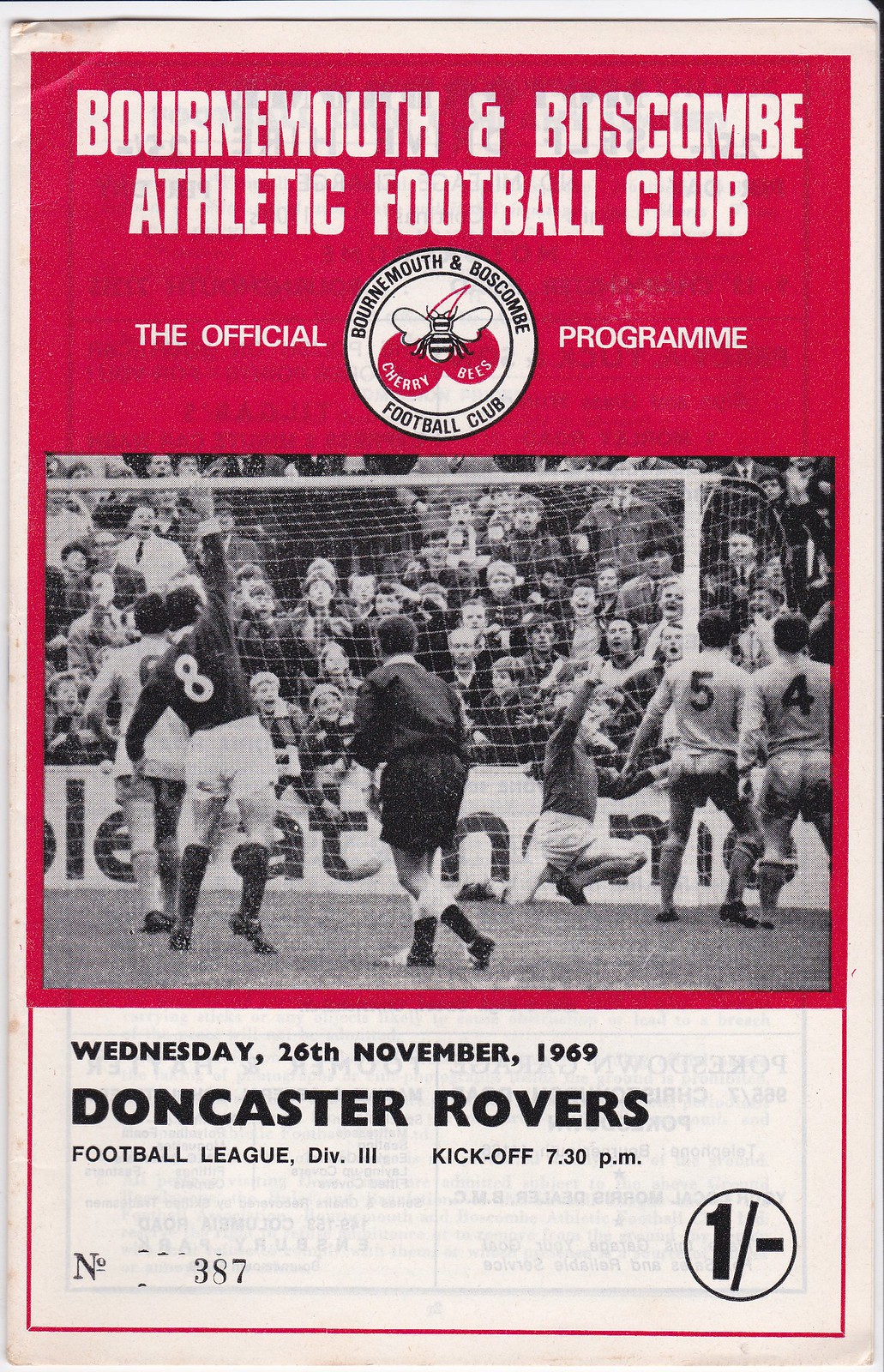This image depicts the cover of a vintage football program from Wednesday, 26th November 1969, featuring a match between Bournemouth and Boscombe Athletic Football Club and Doncaster Rovers in Football League Division 3, with a kickoff scheduled for 7:30 pm. The cover shows signs of aging, with slightly browned edges and small stains. Dominating the top part of the cover is a prominent red text box that states "Bournemouth and Boscombe Athletic Football Club" in white lettering, followed by "The Official Programme." Inside this red section, there is a circular logo featuring an illustration of a bee resting on two cherries, emblematic of the team's nickname, "The Cherry Bees."

Beneath the header, a black and white photograph captures an intense moment of a soccer game in progress. The photo shows players in dark uniforms celebrating, likely after scoring a goal, while others in lighter jerseys exhibit contrasting emotions. The goalkeeper can be seen diving in front of the goal. Behind the action, excited spectators are visible, some standing in anticipation. This program, identified as number 387, originally sold for half a pence, indicated in the bottom right corner.